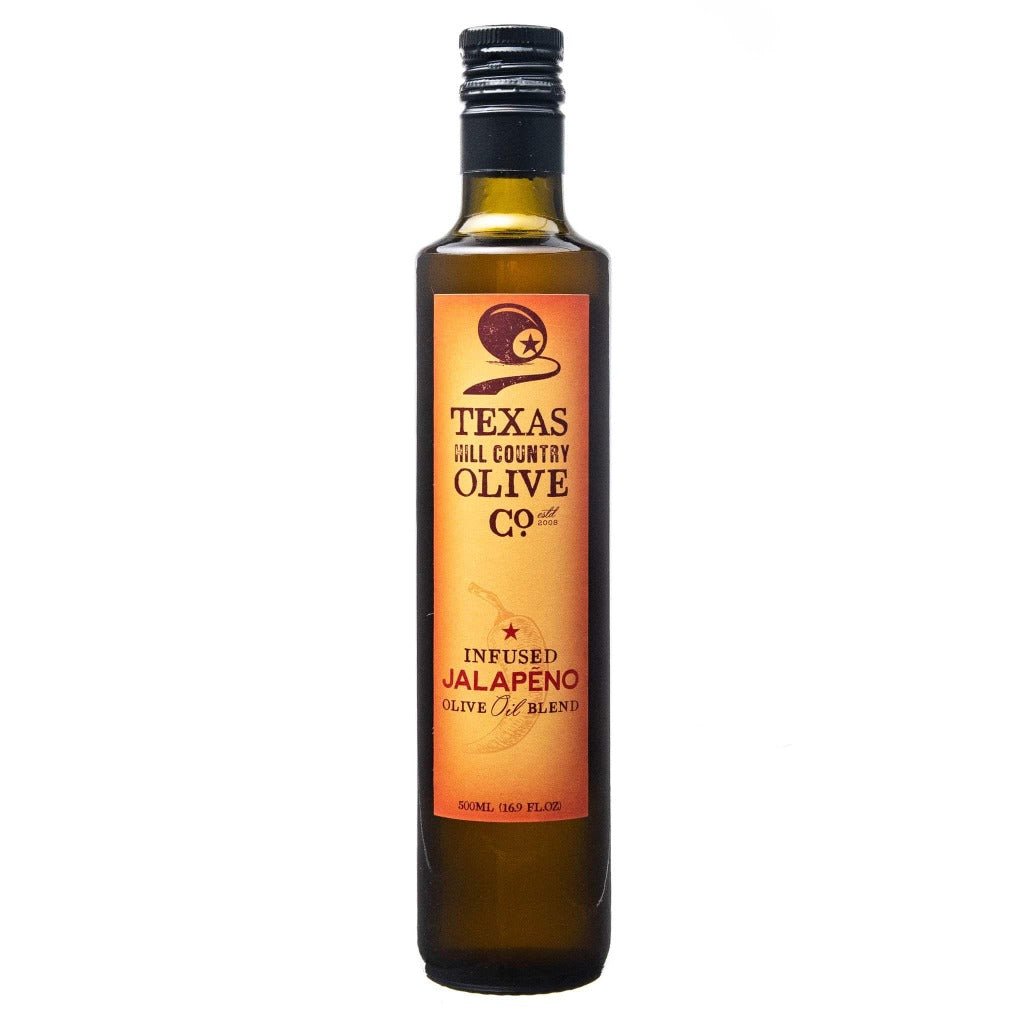The image depicts a tall, slender glass bottle with a greenish-brown hue, reminiscent of an olive. The bottle is topped with a black metal twist-on cap, and the neck features a black rim. The prominent label on the bottle is orange, with a darker orange border and lighter orange center. At the top of the label, there is an illustration of an olive with a star in the pit, which appears to be hanging from a ledge. A winding road-like design emerges from the star. The label reads "Texas Hill Country Olive Co." in bold lettering, followed by "Infused Jalapeno Olive Oil Blend." Towards the bottom, the label displays the volume of the bottle as 800 milliliters or 16.9 fluid ounces. There is also a subtle background image of a jalapeno behind the text.